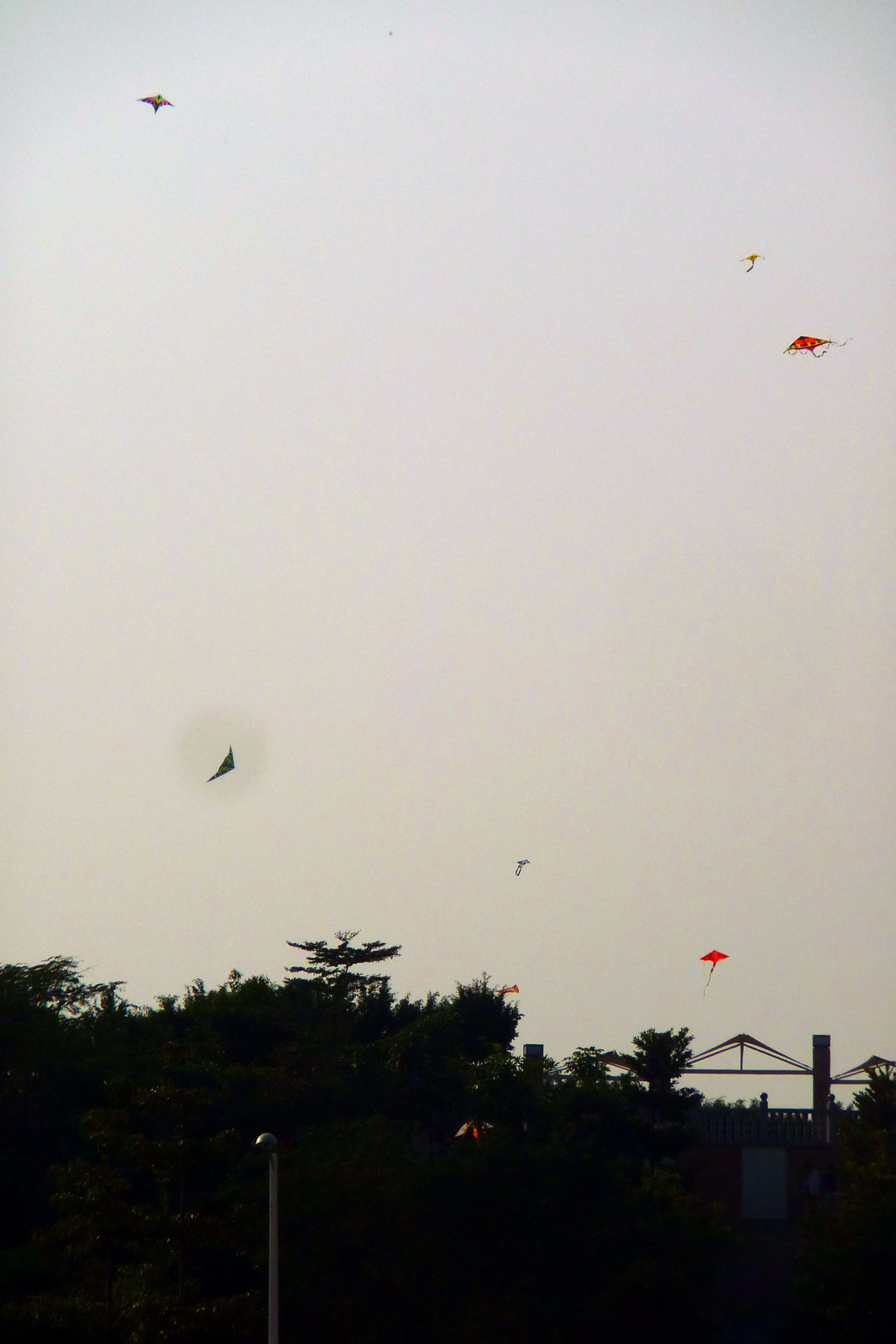The image captures a serene, late evening or overcast sky, occupying the upper half of the frame with six small, triangular kites, some shaped like birds, flying. Below, dark, almost shadow-like trees form a stark contrast, while a bridge with triangular trusses stretches across the right side of the scene, possibly spanning over a dark, indistinguishable river. A large overhead streetlamp stands in the foreground, adding to the quiet atmosphere. The kites, in red and black, seem to be flown by people on the distant bridge, enhancing the image's tranquil and communal feel.